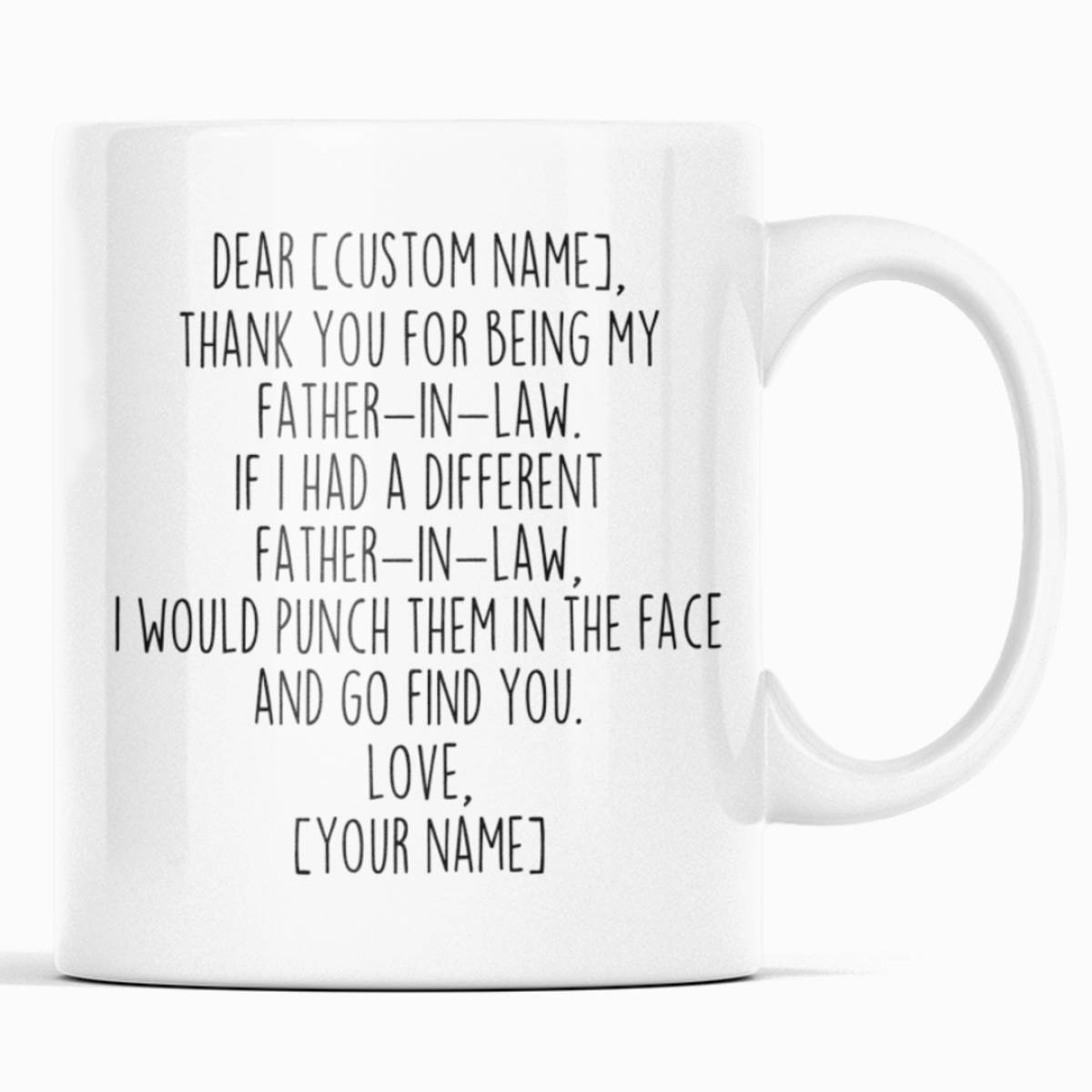This is a detailed photograph of a large, white porcelain coffee mug, showcased against a completely white background. The mug, positioned centrally, features a robust handle on the right side, designed for a comfortable grip. The minimalist design is punctuated by a humorous and affectionate message in bold black text. The message reads: "Dear (Custom Name), thank you for being my father-in-law. If I had a different father-in-law, I would punch them in the face and go find you. Love, (Your Name)." This custom-made mug, ideal for gifting on Father's Day or similar occasions, highlights the capability for personalization with the recipient's and sender's names. The stark contrast of the black lettering against the white mug emphasizes the sentimental and playful nature of the message. The overall aesthetic is clean and modern, with the mug's shadow subtly visible on the surface, adding depth to the image.